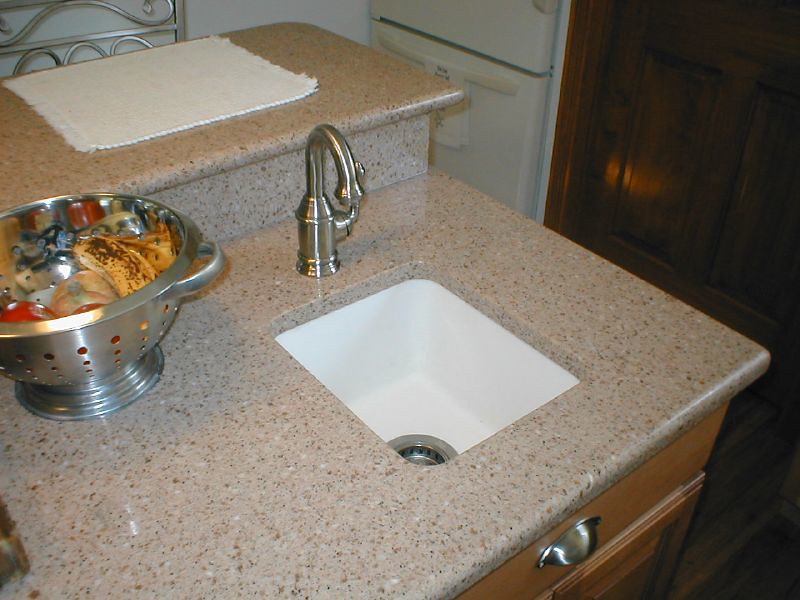In the image, we see a cozy kitchen scene centered around a beige granite countertop. To the right, a sturdy wooden door, likely leading outside, adds warmth to the space. At the end of the counter sits a compact yet deep rectangular sink, presumably for rinsing vegetables and fruit, rather than washing dishes. The sink appears to be made of white porcelain, equipped with a chrome mixer tap featuring a right-side lever.

Adjacent to the sink is a stainless steel colander containing an overripe banana, two onions, and two tomatoes, suggesting the beginnings of a meal prep. Behind the sink and colander, a step-like level leads to a breakfast counter. This elevated counter is set up for dining, evidenced by a white placemat and a partially visible chair. The chair, with its silver wrought iron back, is neatly pushed under the counter.

The kitchen's dark laminated wood flooring contrasts with the light-colored wood cabinetry glimpsed below the counter, creating a warm and inviting atmosphere.